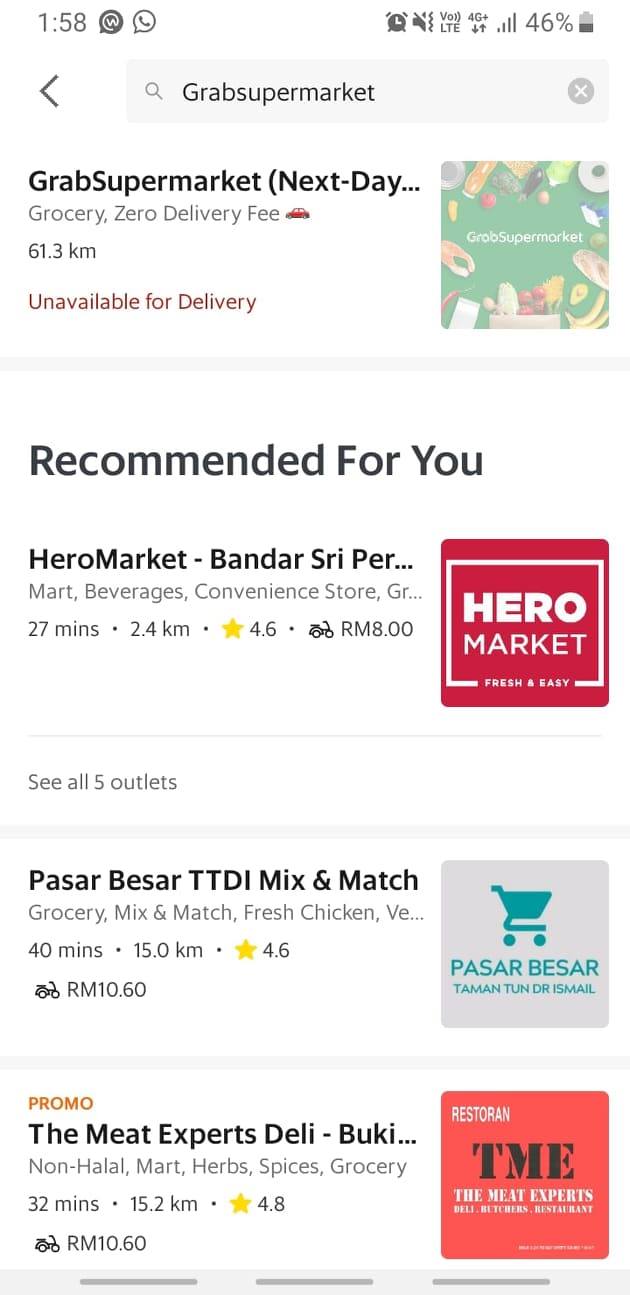The screenshot captures the interface of a cell phone. At the top of the screen, the time is displayed as 1:58 PM. Next to the time, there are two icons: one resembling a phone messenger icon, and another depicting a messenger icon with a 'W' in the middle. The upper right corner shows the alarm icon, the fingerprint (fringer) icon, the full LTE icon (indicating 4G network reception), and a cell phone reception icon. The battery level is indicated at 46%.

Below these icons is a search bar with the text "Grab Supermarket," and just beneath it, the same term appears again, followed by "(next day)" in parentheses, indicating the expected delivery schedule. Further down, the text "Grocery with zero delivery fee" is displayed along with a small car icon. The screen then shows "61.3 KMs," followed by the message "Unavailable for delivery."

Below this, there's a "Recommended for You" section showcasing various markets and delis: Harrow Market, Pasa Besar, and The Meat Experts Deli.